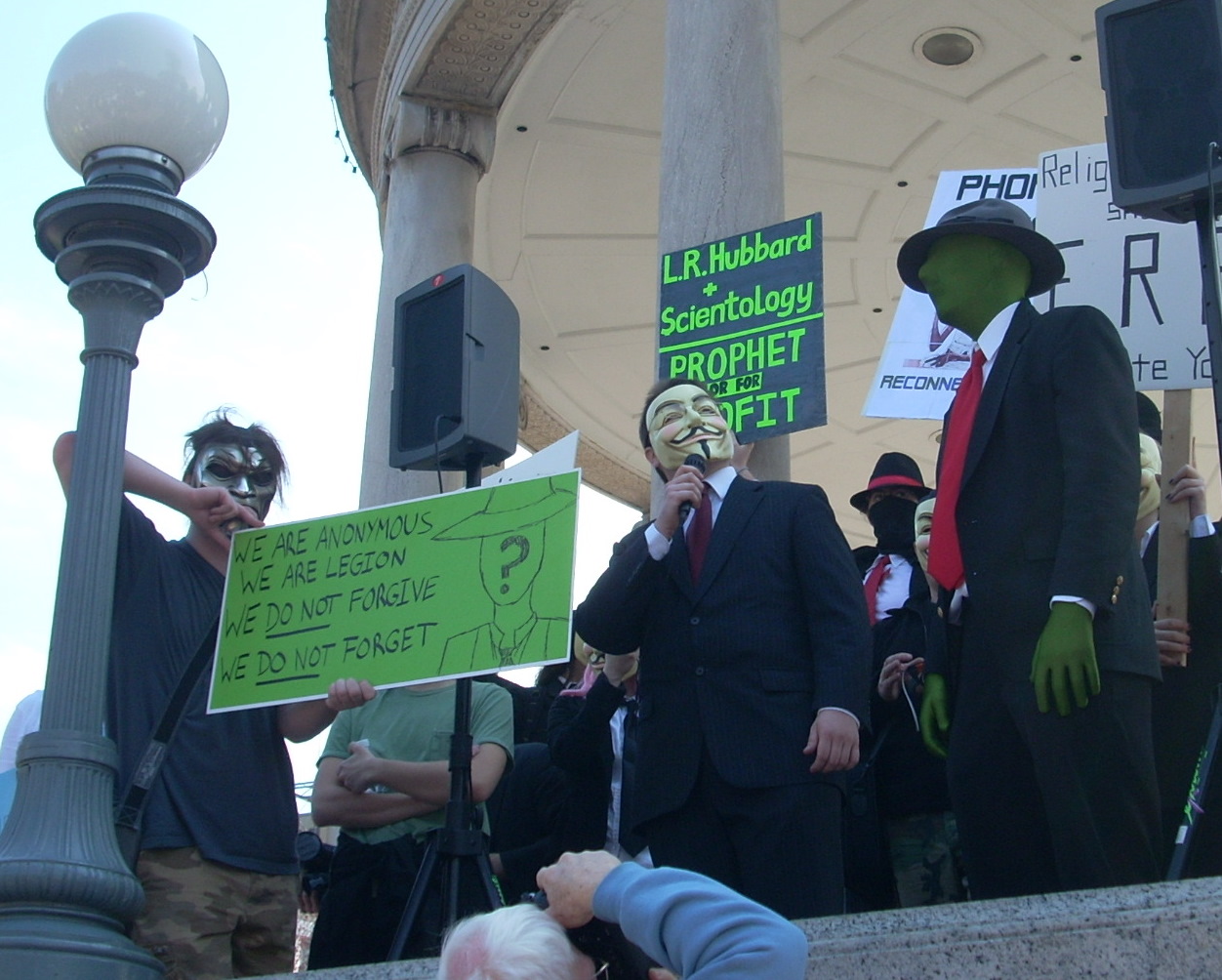In this image, there is a bustling outdoor protest with numerous people wearing masks. The scene is framed by a lamppost with a round bulb on the top, situated to the left of the image. The protesters are gathered in front of a notable round structure with columns, likely somewhere in Boston. The focal point includes a man in the center wearing a suit and an Anonymous mask, famously known from the movie "V for Vendetta." He holds a microphone and stands prominently alongside a sign that reads, "We are anonymous, we are Legion, we do not forgive, we do not forget." 

To his left, a man stands with a similarly worded sign, featuring a detailed drawing of a person with a question mark on his face. Another prominent sign behind the central figure reads, "L.R. Hubbard + Scientology, Prophet," likely indicating a protest against Scientology. To the right of the central figure, a man in a darker green suit, resembling attire used in green-screen special effects, stands out with his suffocated green cloth mask that covers his entire face, including nose and eyes. Additional masked individuals, some in black masks, hold various indistinguishable signs, further contributing to the message of this collective protest.